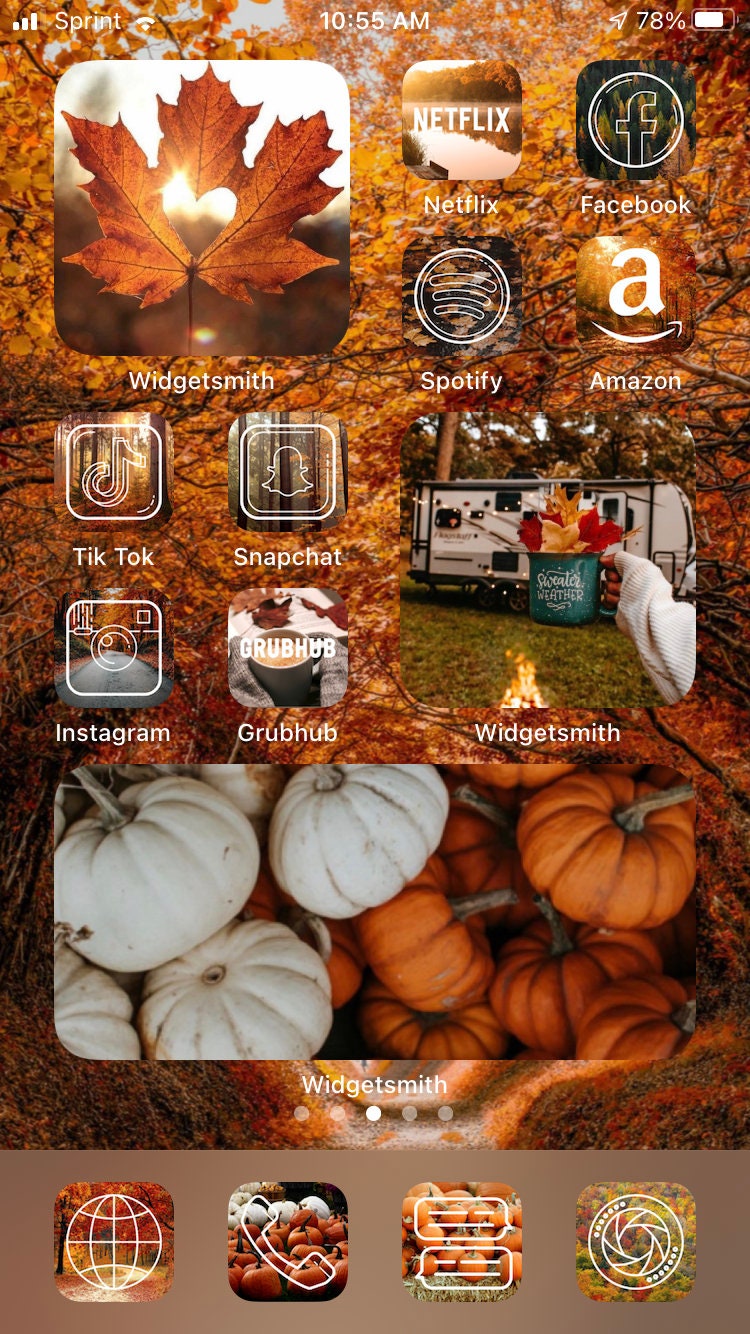A screenshot of a smartphone with a distinctly autumn-themed background is displayed. The top half of the background showcases beautiful fall foliage, featuring vibrant yellow leaves. Below, a cluster of pumpkins can be seen, with the ones on the left being white and the ones on the right being classic orange. The overall aesthetic evokes a cozy autumn feel, reminiscent of pumpkin spice.

The status bar at the top indicates the time is 10:55 AM, with the battery level at 78%. The network carrier is Sprint. The home screen features several app icons, including Netflix, Facebook, Spotify, Amazon, TikTok, Snapchat, Instagram, and Grubhub.

Additionally, there are unique Widgetsmith widgets: one displays a yellow maple leaf with a heart cutout, through which sunlight streams, and another shows a whimsical scene featuring a chicken, possibly near a trailer with a campfire. The meticulous setup exudes a passion for fall and a blend of useful apps, embodying a modern, everyday smartphone setup.